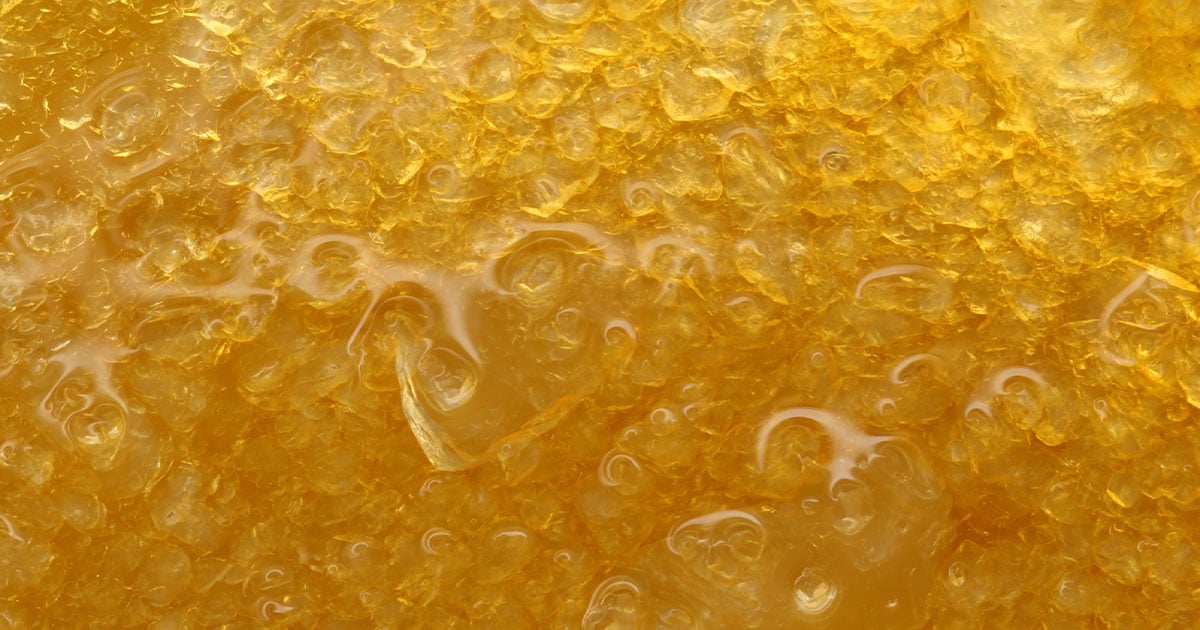This is a detailed color photograph depicting an unclear yellowish gold substance that resembles honey. The substance appears to be contained within a borderless enclosure, suggesting a close-up view that fills the entire frame. Its texture varies across the image, transitioning from a brighter, golden hue at the top to a deeper, more orange shade towards the bottom. The material's consistency seems viscous, reminiscent of honey, as it exhibits both liquid and solid characteristics. Small, smooth areas reflect light, while the rest of the surface is mottled with numerous tiny dips and bumpy structures, likely created by trapped air bubbles. Swirls of white and patterned textures suggest a thick, textured surface, possibly akin to honeycomb. Despite these details, the substance's exact nature remains unknown, with no additional context, text, people, animals, or objects present in the image to provide further clues.